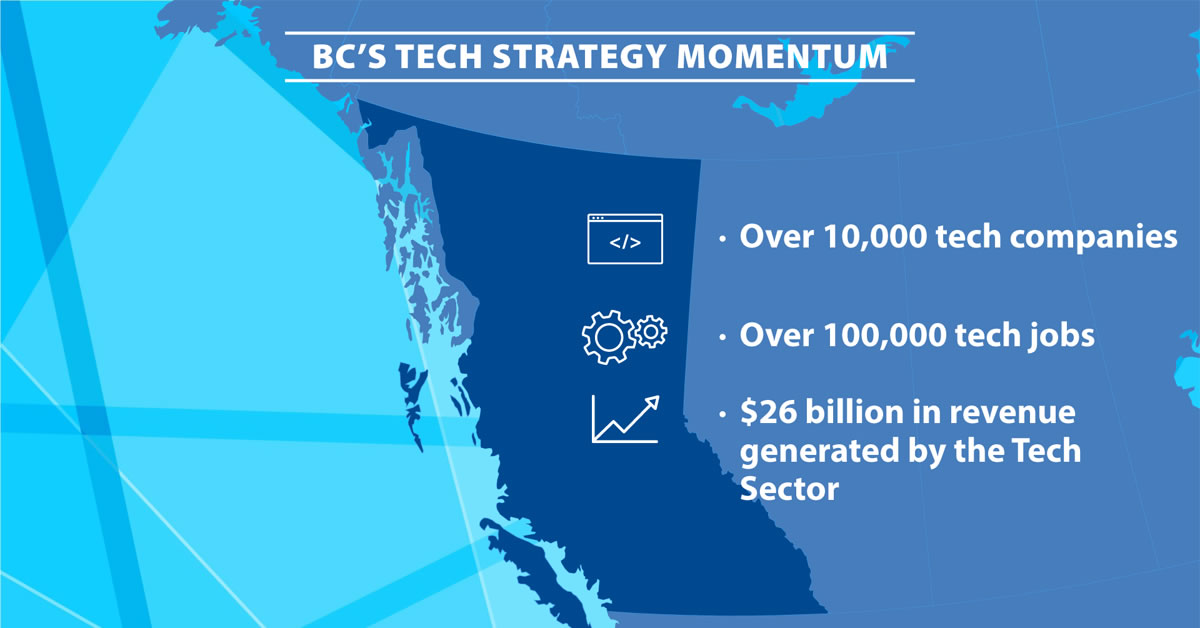The image is an advertisement for a company's mission, titled "BC's Tech Strategy Momentum," featured predominantly at the top in bold, white capital letters, encased by horizontal lines above and below. The background is predominantly blue with varying shades creating an abstract landscape that might resemble a map. It showcases a medium blue color with a darker blue shape near the center and a lighter blue area on the left with a window pane pattern overlay. Integrated are three descriptive bullet points each accompanied by a white line art icon to its left. The first bullet point, alongside a small graphic, highlights "over 10,000 tech companies." The second bullet, marked by two small gear icons, states "over 100,000 tech jobs." The third bullet, accompanied by a charted arrow icon, declares "$26 billion in revenue generated by the tech sector." The text and icons are all in white, designed in an information graphics style that combines illustration and typography for a clear and compelling visual.